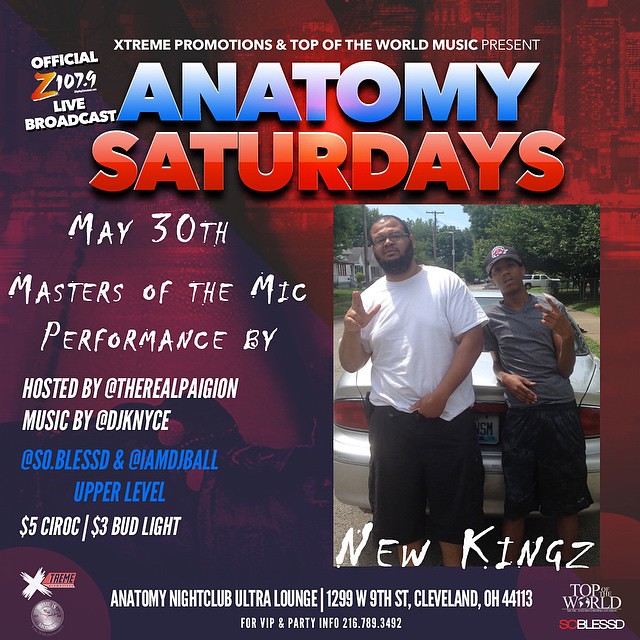An official Z107.9 live broadcast advertisement for "Anatomy Saturdays" at the Anatomy Nightclub Ultra Lounge in Cleveland, Ohio. The event, taking place on May 30th, features the "Masters of the Mic" performance, hosted by The Real Pagean, with music by DJ Canice. The ad highlights special drink prices of $5 for Chirac and $3 for Bud Light. The vibrant, colorful design incorporates blue, red, black, and white lettering. In the foreground of the image, two African American gentlemen, one portly wearing a white shirt and black shorts, the other slightly smaller in a gray shirt and black shorts, pose for the camera, making hand gestures that appear to mimic gang signs. They are leaning against an indistinguishable gray car with trees visible in the background. The nightclub is located at 1299 West 9th Street, Cleveland, Ohio, 44113. For VIP and party information, the contact number is 216-789-3492.